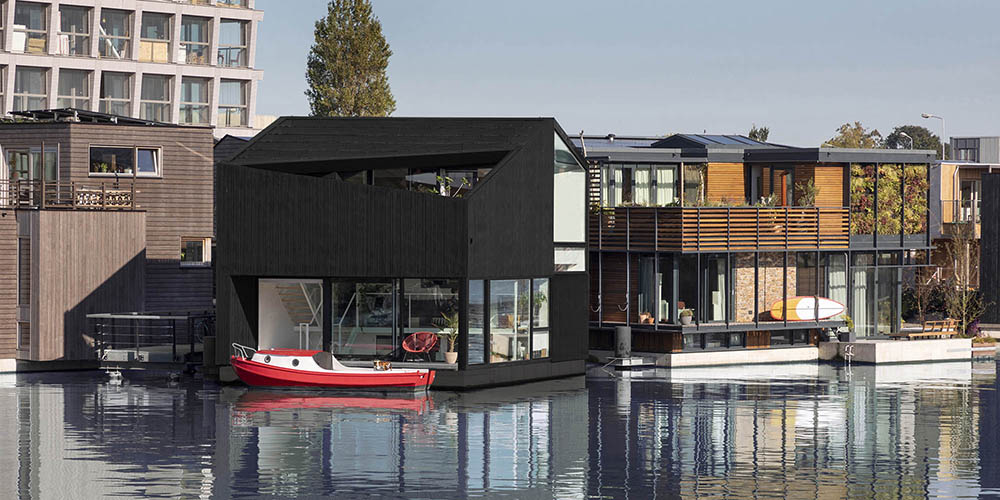This detailed photo captures a picturesque waterfront scene featuring an eclectic mix of houseboats and lakeside homes. Dominating the image is a sleek, black modern house with large picture windows and a red chair outside, reflecting elegantly in the calm water. Adjacent to it is a rustic brown boathouse with a combination of brick and metal elements, exuding a log cabin-like charm. Alongside these, another smaller brown house and a beige building set further back from the water complete the lineup of structures. A red speedboat with white-trimmed windows is prominently parked in front of the black house, adding a splash of vibrant color to the scene. The tranquil setting is enriched by a large green tree standing in the background against a clear blue sky, suggesting a beautifully serene and sunny day. The area exudes a relaxing, almost tourist-like ambiance, perfect for soaking in the natural beauty of the lake.